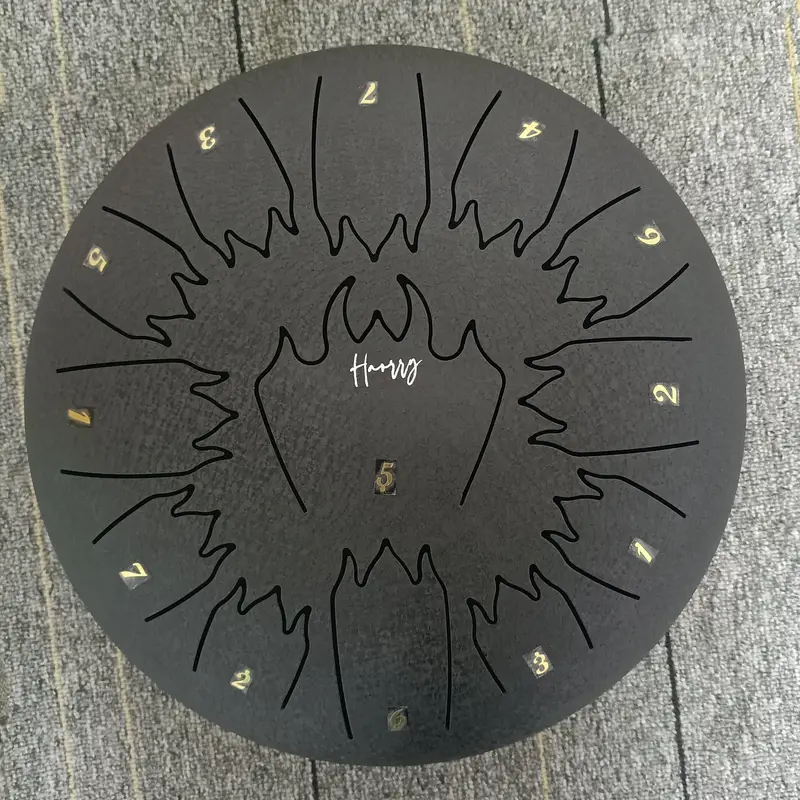In the image, an overhead view captures a dark gray, circular disc set against a light gray background, possibly a carpet or table. This object, possibly a clock, sundial, or decorative plate, exhibits a series of gold or yellow numbers arranged in an unconventional sequence around its perimeter: 1, 5, 3, 7, 4, 6, 2 at the top, and 7, 2, 6, 3, 1 at the bottom. The center of the disc features the number 5 amidst a striking black outline of a devilish or bat-like figure with horns and spiky elements. Surrounding this central design are black line drawings resembling spiked creatures, all pointing inward. The image uses a muted palette including shades of gray, black, beige, and touches of white, focusing on the disc from a top-down perspective. The setting and purpose of this object remain ambiguous, adding to its intriguing nature.